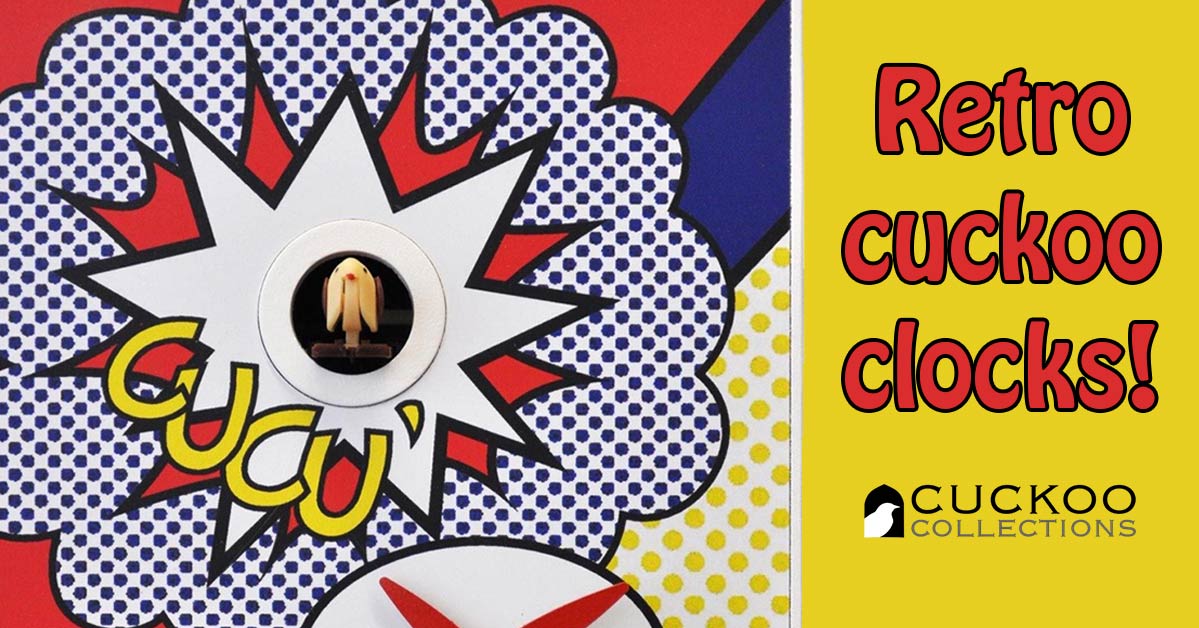This vibrant and artistic advertisement for Retro Cuckoo Clocks captures attention with its comic book-style design and bold coloring. The right side of the image features a gold background with robust red text proclaiming "RETRO CUCKOO CLOCKS!" Below it, "CUCKOO COLLECTIONS" is displayed in black lettering, next to an emblem consisting of a white bird set against a black backdrop. Dominating the left side is an intricate op-art-themed design, featuring a blue and white polka dot pattern on a red and blue striped background. At the center of this left section is a dramatic white burst emanating from a red burst, outlining a photograph of a white dog with long floppy ears, resembling a stuffed animal. Below this central image is the word "CUCÚ," written in lively yellow font. This whimsical and engaging ad bridges vintage charm with modern graphic design flair.